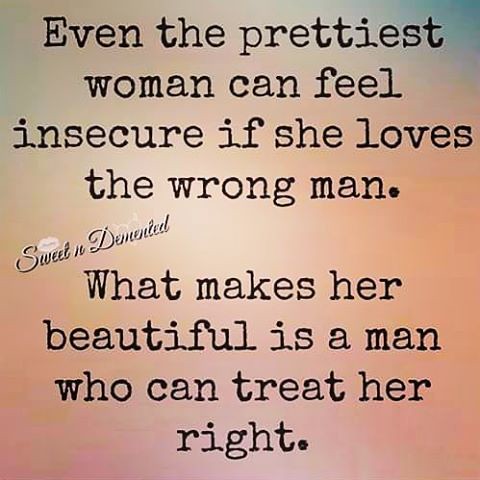This square computer graphic features a softly blended background of light orange, pink, and blue, creating a demure, cloud-like pattern. Over this aesthetically pleasing gradient, the text is prominently displayed in a typewriter-like, black font. The text reads, "Even the prettiest woman can feel insecure if she loves the wrong man. What makes her beautiful is a man who can treat her right," formatted in two clear sentences, giving it a thought-provoking impact. Positioned diagonally in a script font in the middle, slightly leaning to the right, is a signature or watermark that reads, "sweet and demented." This graphic combines a visually soothing design with a meaningful quote, making it suitable for framing on a wall or sharing on social media.